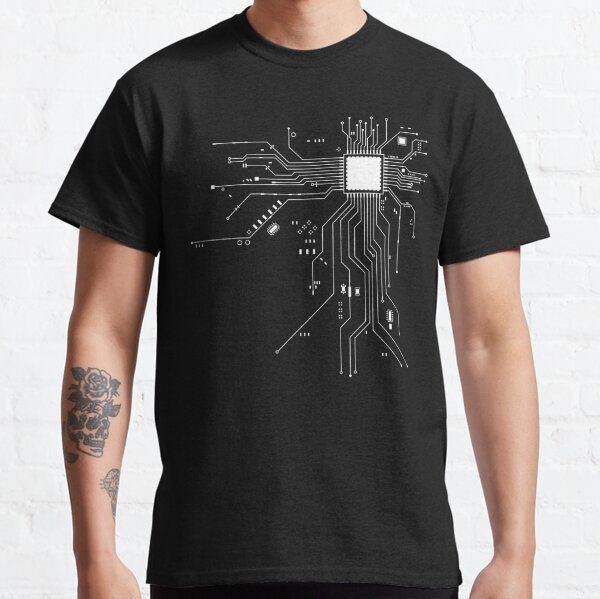The image showcases a Caucasian man modeling a heathered charcoal-black, short-sleeve, crewneck t-shirt against a soft white brick wall. The t-shirt features an intricate design resembling computer circuitry, prominently displayed on the left side of his chest, interwoven with what looks like a white square amidst the pattern of wires. The man's right arm is adorned with a detailed tattoo of a rose, extending down to his inner wrist area. His skin tone is warm but not particularly tan. The photograph, likely intended for print-on-demand purposes, puts a strong emphasis on the contemporary tech-inspired t-shirt design.